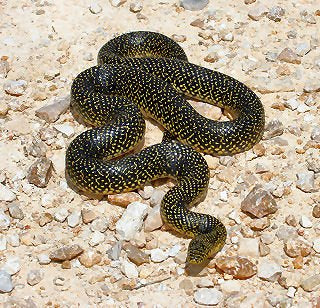The image is a low-quality, slightly out-of-focus outdoor photograph in a square format. It captures a snake centrally positioned on a rough, rocky terrain. The ground features a mix of large rocks and stones in shades of light tan, white, grey, and brown. The snake, which is a striking black on its upper side with white speckly detailing, has its head facing towards the camera, although the shot is taken from a higher angle looking down. The underside of the snake, in contact with the ground, exhibits a yellowish tinge. The snake's body is coiled in S-shapes, with its tail tucked underneath, yet all parts of the snake are visible within the frame.